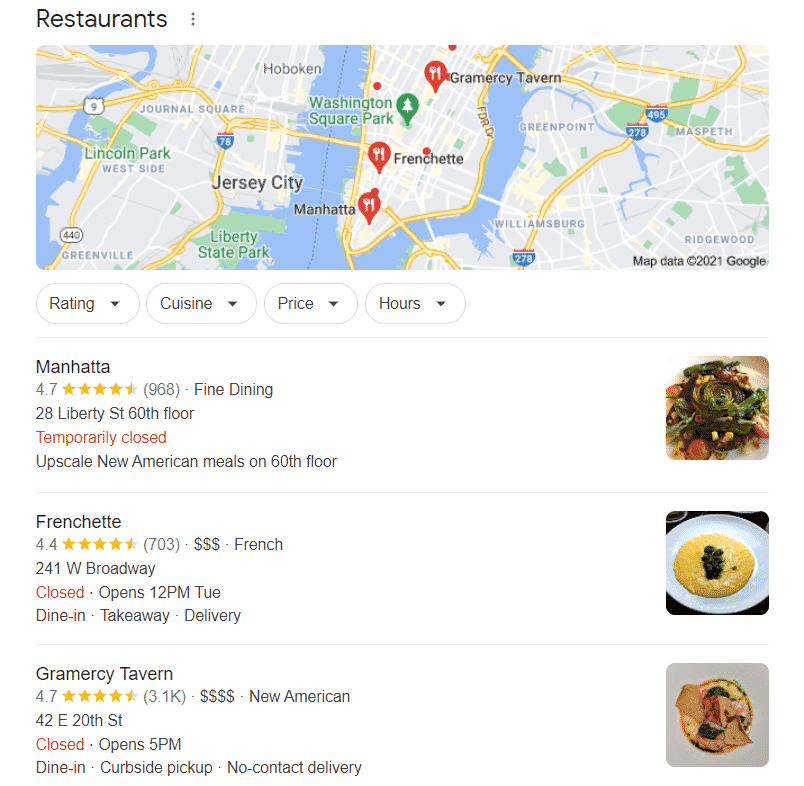This is a detailed map of Manhattan featuring three red balloons, each marked with a fork and knife to denote restaurants.

1. **Manhattan**: Rated 4.7 stars, this upscale dining establishment offers fine American meals on the 60th floor. However, it is currently temporarily closed.

2. **Frenchette**: This French restaurant, located at 241 West Broadway, holds a 4.4-star rating. With a price indicator of $3 bills, it is on the expensive side. Currently closed, it reopens at 12 PM on Tuesday and offers dine-in, takeaway, and delivery options.

3. **Gramercy Tavern**: Situated at 42 East 20th Street, Gramercy Tavern boasts a 4.7-star rating and serves New American cuisine. It is known for its higher price range, denoted by $4 bills. The restaurant is presently closed and will reopen at 5 PM, offering dine-in, curbside pickup, and no-contact delivery services.

Additionally, the map includes images of dishes from each restaurant, providing a visual taste of what to expect.